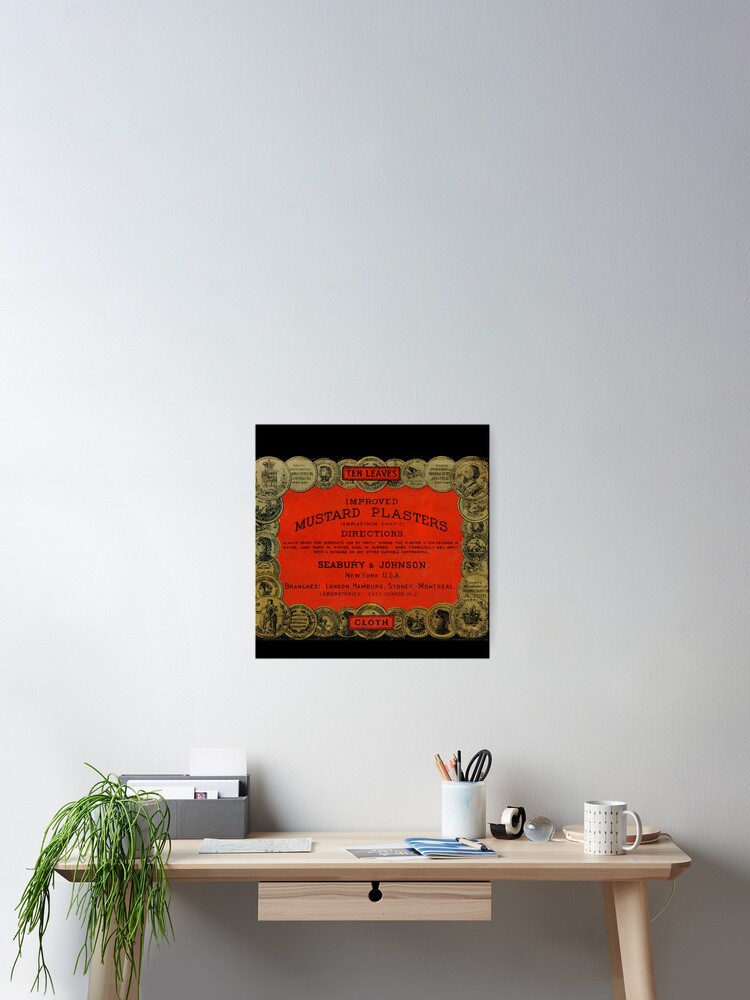The image showcases a home office setting with a light beige wooden table. The table has outward-extending legs and is adorned with various items, creating a somewhat cluttered appearance. Among the items on the table are a white cup holding pens, a gray container filled with scissors and pins, a small white desk lamp situated on the right side, and a green plant that appears either wilted or hanging off the side. Additionally, there are various papers scattered on the table. In the background, dominating the scene, is a large sign or poster featuring what seems to be a recreation of an old-time advertisement in vibrant reddish-orange and black text on a black background. The sign reads "Improved Mustard Plasters" followed by "Seabury & Johnson, New York, USA," and possibly other text that's difficult to discern due to its small size. The entire setup suggests a blend of minimalistic and vintage decor elements within the home office space.